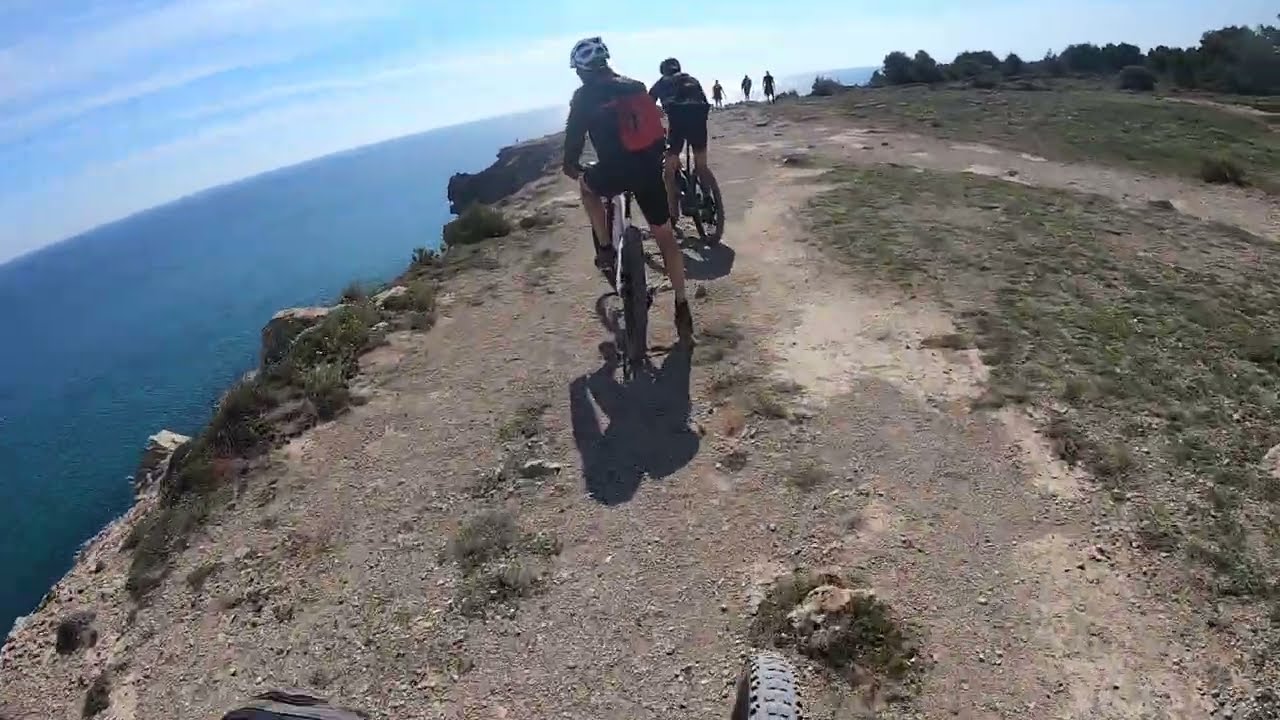This outdoor photograph, taken from a wide angle, captures a sunlit, cliff-top scene overlooking a blue ocean to the left. The sky is mostly clear with fluffy white clouds. The ground is a mixture of dirt, rocks, and sparse vegetation, with little sprouts of grass scattered about. Dominating the center of the image are two mountain bikers, seen from behind, wearing helmets, backpacks, and bicycle shorts. Their thick, wide tires suggest they are prepared for rugged terrain. They appear to be gazing towards the ocean. A front bike tire at the bottom of the image suggests another cyclist is just behind them. Further along the rocky, gravel-strewn path, three people can be seen walking. To the right, a tree line marks the beginning of a wooded area. This vibrant nature scene exemplifies a perfect day for outdoor exercise and exploration.